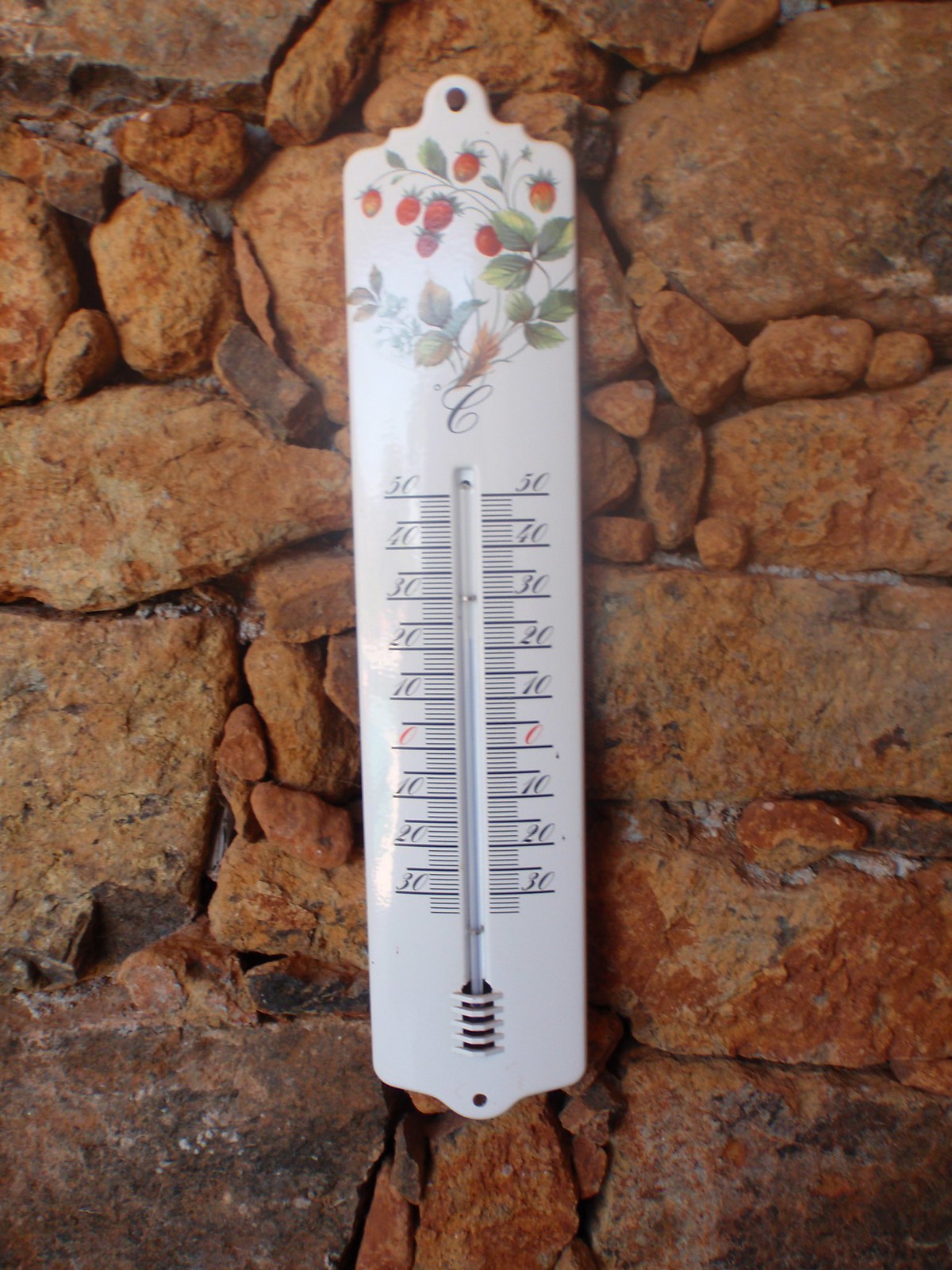A tall and narrow white metal mercury thermometer is mounted on a stone wall using a nail secured through a hole at the top. The thermometer features a central glass tube filled with mercury, flanked on both sides by black hash marks and numbers. The numeric scale begins at 30 at the bottom, descending to 20, 10, and 0, then ascending from 10 to 50, with the zero uniquely highlighted in red. At the top of the thermometer, there are decorative elements including painted leaves and strawberries, adding a touch of charm to the functional device.